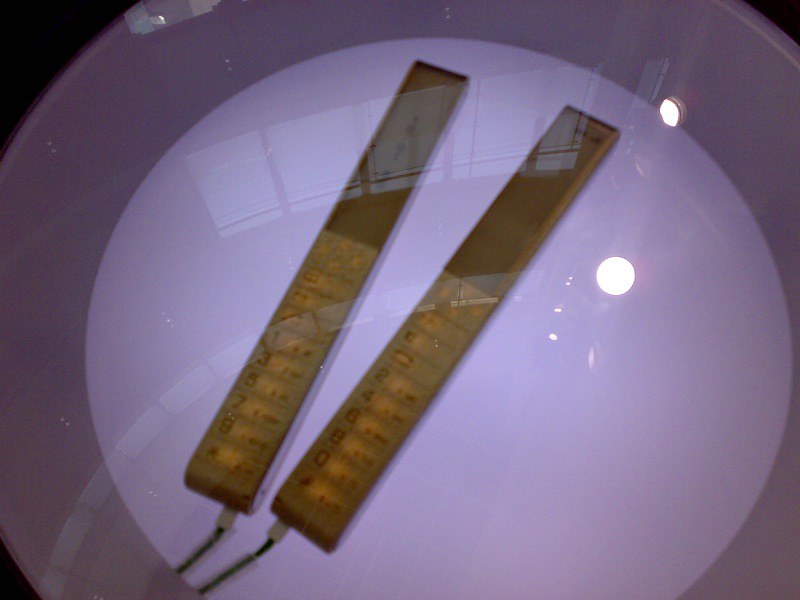The image features two long rectangular objects placed on a highly reflective surface, likely under glass, which captures reflections from surrounding lights and possibly a window. These objects rest on a plate with a white center and a gray rim. The rectangles resemble brown sticks or bars with darker tops and are attached to what appear to be fuses, wires, or cords. The bottoms of these rectangles transition to a lighter brown and display numbers in red. The first rectangle on the left shows numbers 1, 3, 5, 7, and 8. The second rectangle on the right displays numbers 2, 4, 6, 8, and 0. Additionally, there may be other symbols, like a star and pound key, but they are not clearly visible.